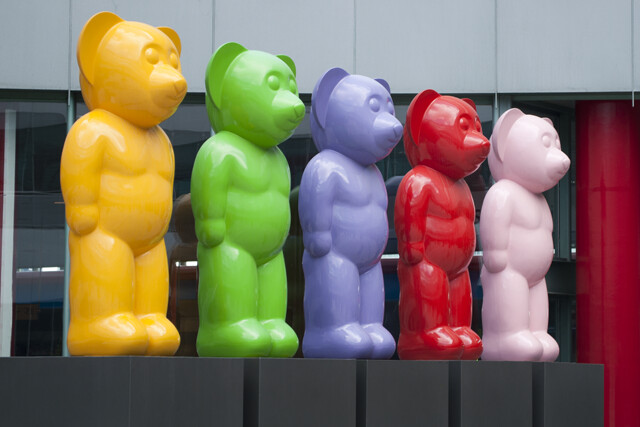The image captures a vibrant row of five multicolored teddy bear statues, which seem to be made out of shiny, high-gloss plastic, standing on a black surface indoors. These bears are human-like in their upright posture, with round ears, pointed noses, large round eyes, and smiling mouths, all facing slightly to the right. From left to right, the bears are colored dark mustard yellow, bright lime green, lavender purple, bright strawberry red, and baby pastel pink. The backdrop is gray with a red pole on the right, adding a touch of contrast to the scene, which may be part of a building’s interior decor. The photograph, noted for its excellent quality and detail, captures these cheerful figures in a playful arrangement.